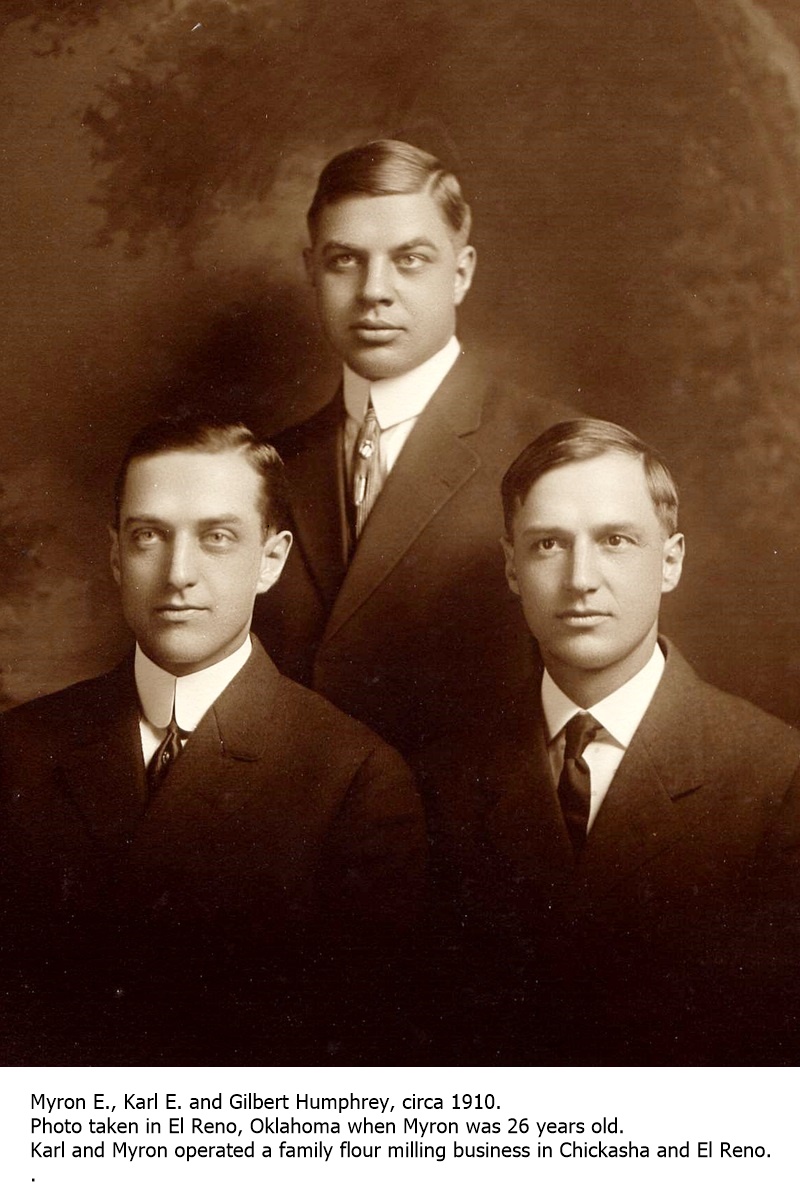This antique sepia-toned photograph, dating from around 1910, captures three young men in their mid-20s. The image has a warm brown hue typical of sepia, rather than traditional black-and-white monotones. Central in the back is a gentleman with a slightly rounder face and prominent eyebrows, looking off-camera with a particularly serious expression. In the foreground, two more men are seated, also dressed in dark suits paired with white button-up shirts and ties. All three share similar hairstyles, with dark hair neatly parted to the right. They pose against a neutral photographic backdrop with indistinct splotches, adding some contrast and depth to the scene. Below the image, a caption reads: “Myron E., Carl E., and Gilbert Humphrey circa 1910, photo taken in El Reno, Oklahoma when Myron was 26 years old.” It also notes that Carl and Myron operated a family flour milling business in Chickasha and El Reno.